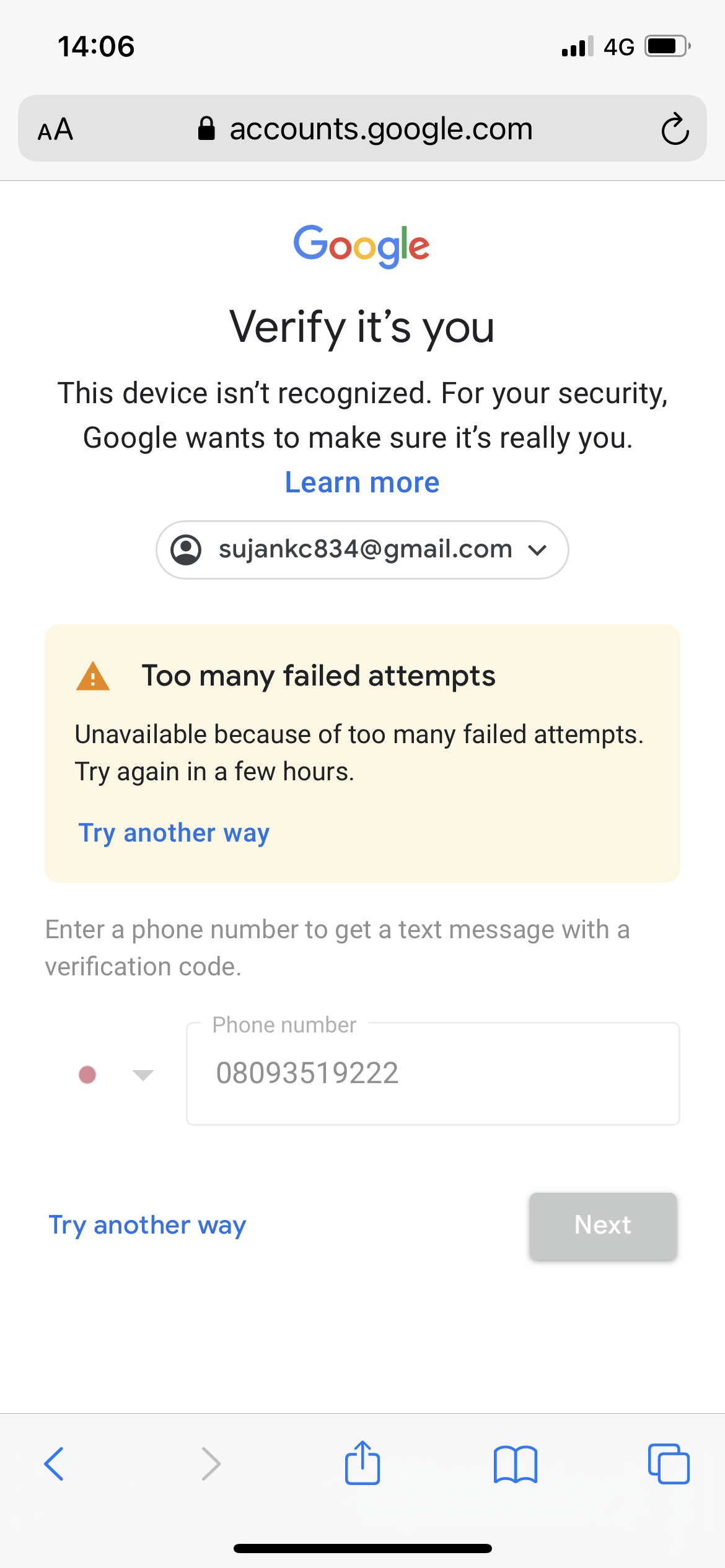This is an image captured from a mobile phone screen, displaying a notification from Google. At the top of the screen, the time reads 14:06. The upper-left corner shows a signal icon, while the upper-right corner indicates the battery status at approximately 75% along with the "4G" network symbol and the Wi-Fi signal bars.

Beneath this, there are two overlapping 'A' icons within the search bar area, next to a lock icon displaying the URL "accounts.google.com" and a refresh arrow icon.

The main portion of the screen features Google's logo in colorful letters followed by a security verification message: "Verifying it's you." A smaller font underneath states, "This device isn't recognized. For your security, Google wants to make sure it's really you." Below this message, a blue link reads "Learn more."

Further down, a bar displays an email address, and below that, inside a yellow rectangle, is an alert message. The alert, marked by an orange triangle with an exclamation point, reads: "Too many failed attempts. Unavailable because of too many failed attempts. Try again in a few hours." At the bottom, there is a "Next" button intended for navigation.